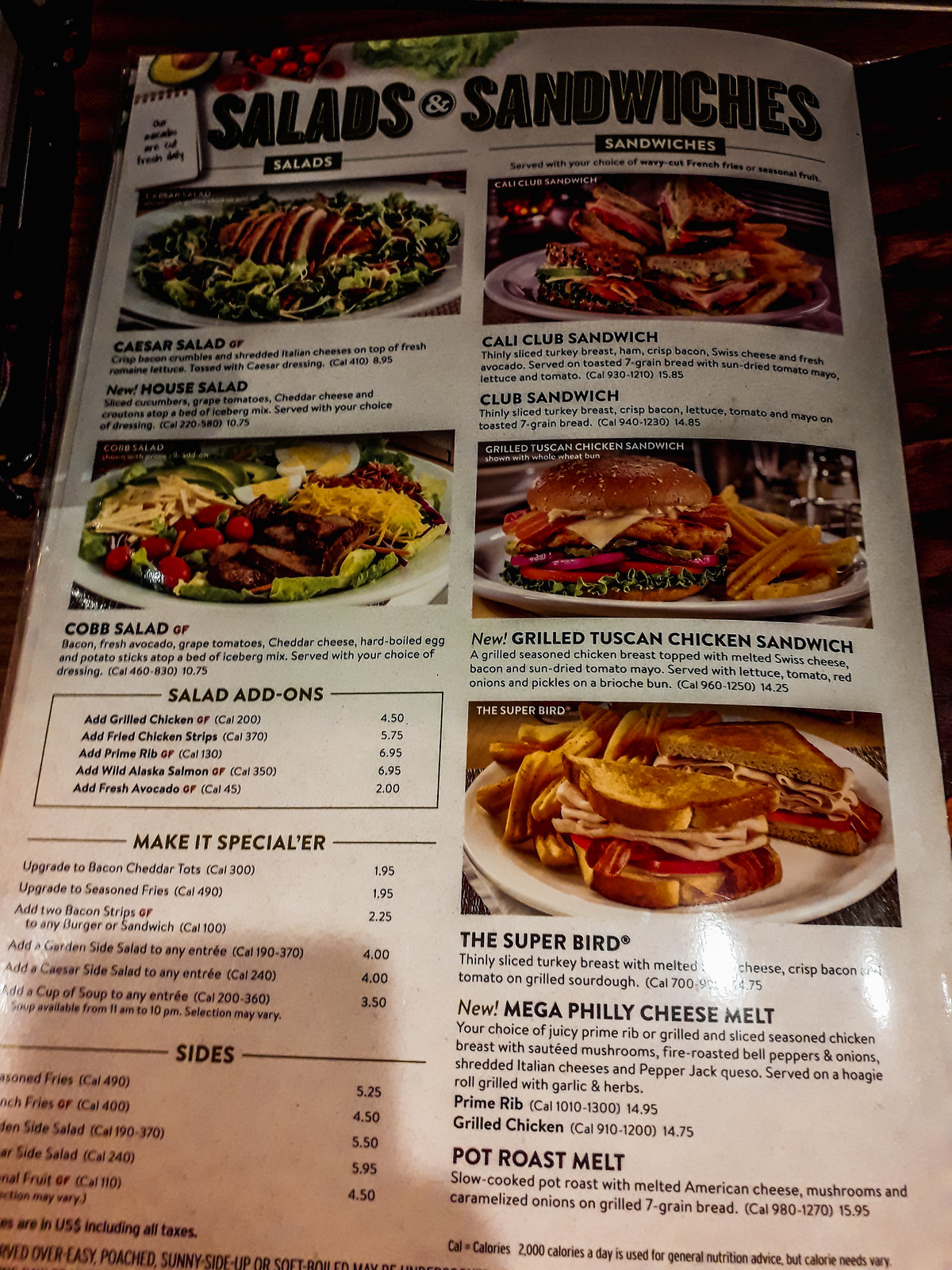The image depicts a menu rich with vivid visuals and detailed descriptions of various salads and sandwiches. Although the name of the restaurant is not indicated, the enticing options are clearly laid out to cater to diverse tastes.

At the top of the menu, the titles "Salads" and "Sandwiches" prominently organize the selections. On the left side, a tempting photograph of a salad crowned with what appears to be grilled chicken captures attention. Below this image, a variety of salad options are listed:

- **Caesar Salad:** No picture provided, presumably includes classic ingredients.
- **House Salad:** Accompanied by a description detailing its components.
- **Cobb Salad:** There is an accompanying photo showcasing greens, cheese, eggs, bacon, and avocado.

Further below, the menu highlights additional toppings available for customization:
- Chicken Strips
- Grilled Chicken
- Prime Rib
- Salmon

The menu also lists extra options to enhance the salads such as cheddar cheese and fries. Finally, the different available sizes of the salads are mentioned.

On the right side of the menu, the focus shifts to an array of sandwiches. Among these are:
- **Cali Club Sandwich**
- **Club Sandwich**
- **Grilled Tuscan Chicken Sandwich:** Featured with an appetizing picture.
- **Omega Philly Cheese Melt**
- **Pat Rose Melt**

A photograph of a club sandwich is also presented alongside detailed descriptions of the sandwich offerings.

In essence, the menu not only provides an array of appetizing choices but also ensures clarity and visual appeal to guide diners in their selections.